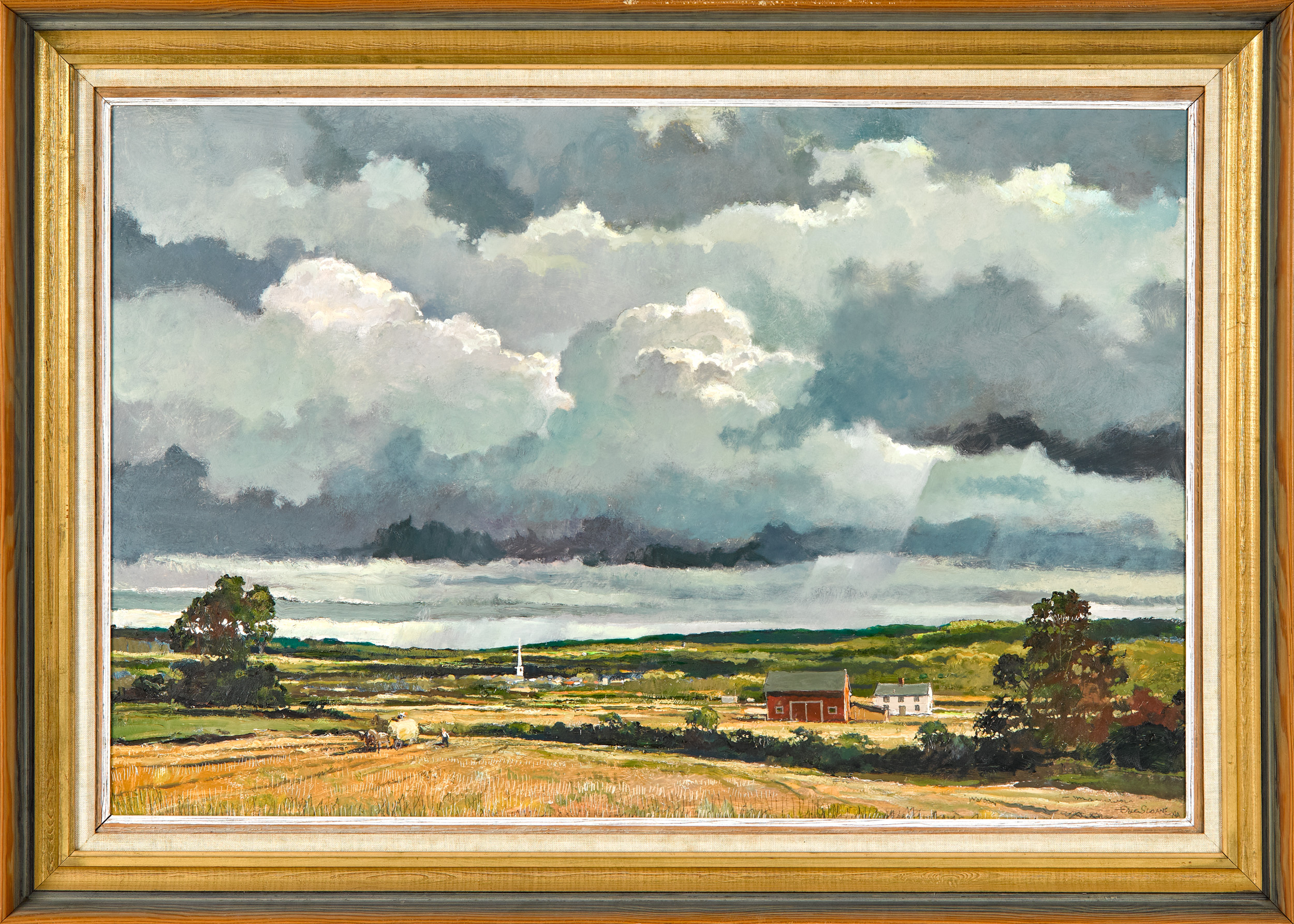The photograph captures a beautifully framed painting depicting a vast landscape dominated by a farm scene. The frame itself features multiple layers: the outermost edge is a dark, burnt-looking brown wood, followed by a lighter brown and then an even whiter wood leading up to the painting. This intricate framing, with four to five distinct colors, complements the detailed artwork within.

The painting showcases a large, tilled field in the foreground, where a bull is harnessed to a wagon, surrounded by people, suggesting active farm work. To the left, partially towards the middle, stand a couple of big green trees, while a green and orangish tree graces the right side. Dominating the center of the landscape is a boxy red barn with white trim, accompanied by a white farmhouse behind it. The sky, occupying about two-thirds of the upper portion, is painted with light grey, blue, and black clouds, conveying an impending rainstorm.

In the background, several buildings cluster together, presumably forming a town, highlighted by a church steeple rising above them. The lower portion of the painting also features a grassy field with tan-colored grass, hinting at a wheat-growing area. Overall, the harmony of colors and intricate details draw the viewer into the rustic charm and serene ambiance of farm life, set against the backdrop of a dynamic sky.